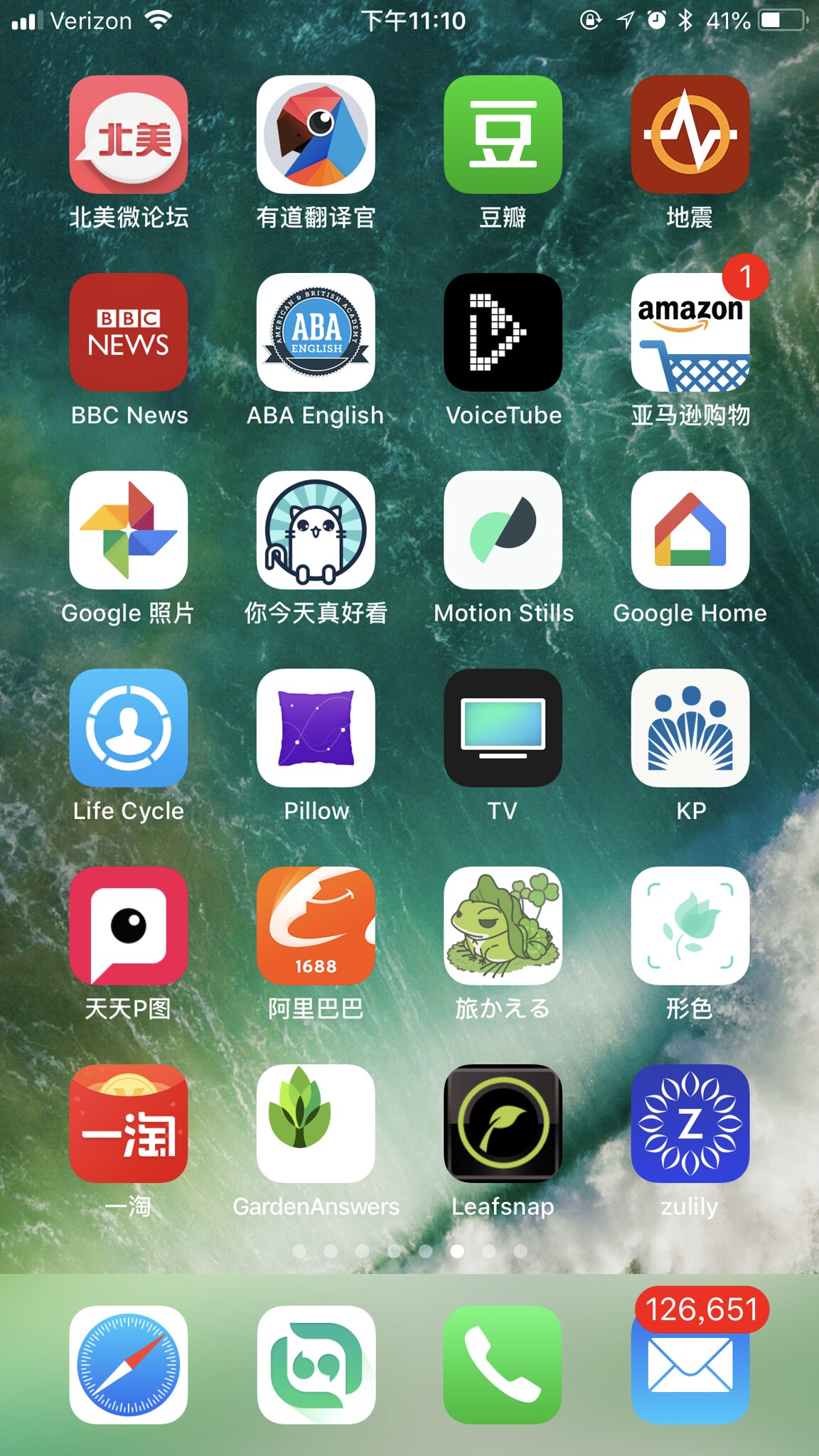The image depicts the home screen of an iPhone belonging to an individual who uses Asian language characters, likely indicating the person is either from or has affiliations with an Asian region. The screen is cluttered with a multitude of app icons, with no folders to organize them, suggesting a high level of app usage or varied interests. There are recognizable apps such as BBC News, Amazon, Lifecycle, and Google Photos amidst numerous apps with Asian character descriptions. The mail icon stands out with an overwhelming 126,651 unread messages. The status bar shows that the phone is connected to Verizon and Wi-Fi, with the current time being 11:10 AM and the battery at 41%. The device is also connected to Bluetooth. The layout hints that the user can swipe through several more pages of apps.